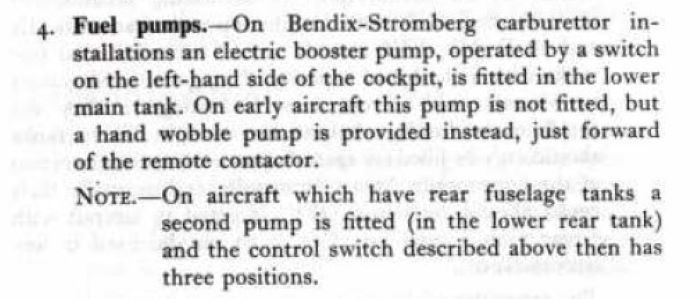The image is a rectangular clipping from a textbook or manual, with a white background and black printed text. It begins with the number "4." followed by "FUEL PUMPS" in bold. The text then describes, "On Bendix Stromberg carburetor installations, an electric booster pump, operated by a switch on the left-hand side of the cockpit, is fitted in the lower main tank. On early aircraft, this pump is not fitted, but a hand wobble pump is provided instead, just forward of the remote contractor." At the bottom, it notes, "On aircraft which have rear fuselage tanks, a second pump is fitted in the lower rear tank, and the control switch described above then has three positions."